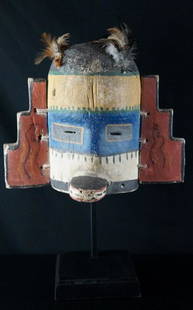Against a completely black background, this color photograph features a museum-displayed mask, possibly of Native American origin, specifically resembling a kachina mask, although some elements hint at diverse cultural influences. The mask, mounted on a black pedestal stand, appears ancient and handmade, likely from organic materials such as leather or tree bark. The head of the mask is domed and topped with feathers, combining black, white, brown, and gray tones. The mask's body is divided into horizontal bands: a top band that is a dark, dirty green; followed by a broad yellow stripe, a blue stripe with gray rectangular eye outlines and small black slits for eyes, a whitish-gray band with thin black lines, and a gray band at the bottom. The mask also features an oval, tongue-like protrusion at the very bottom, edged in a grayish-red outline. On either side of the mask, three-stepped, stair-like red flaps extend outward, secured by cord or similar fastenings.